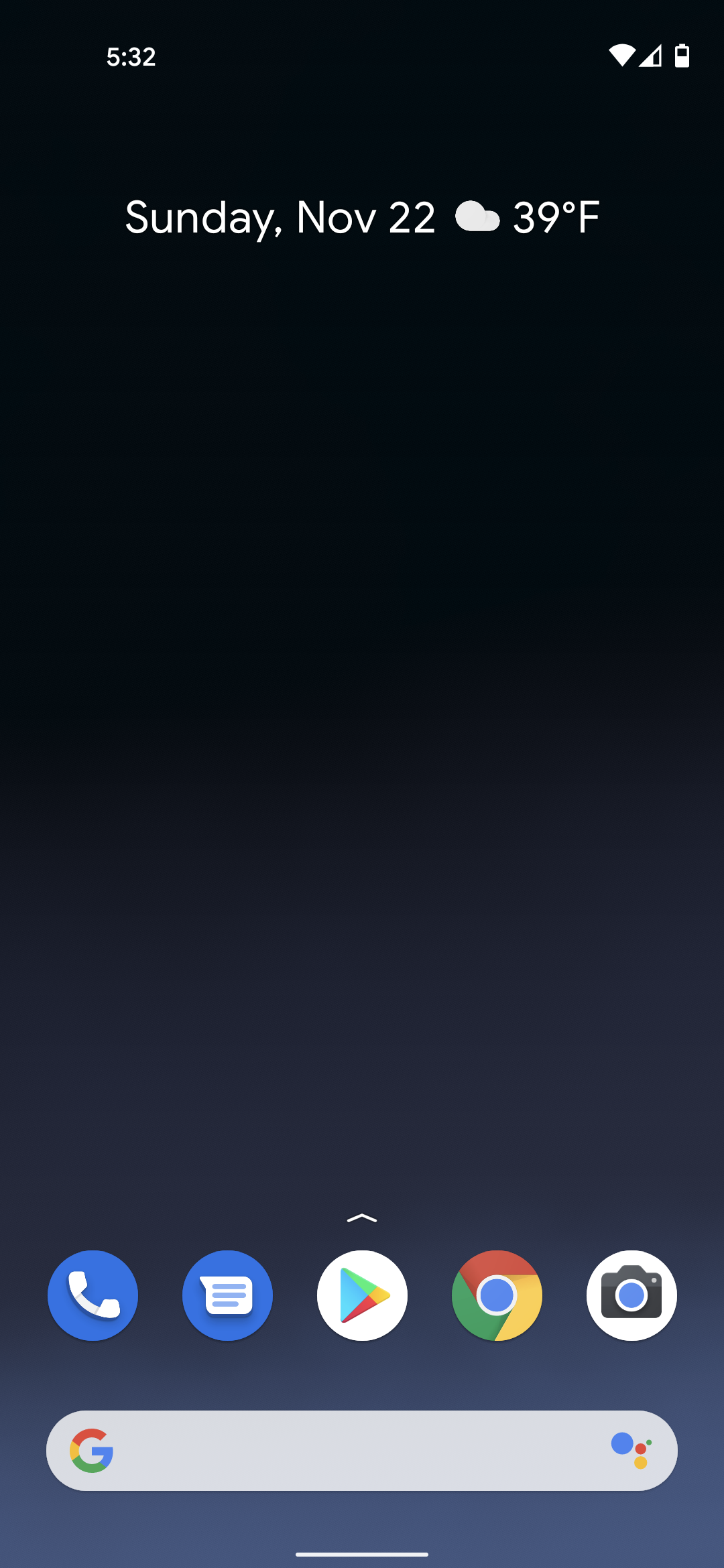The screenshot captures the home screen of a mobile device. The background features a gradient transitioning from blue to black. 

At the top, the status bar shows the time on the left as 5:32 and the battery level on the right at 75%. Below the status bar, the screen displays the weather information with "Sunday, November 22nd," a cloud symbol, and the temperature reading "39°F."

Centered on the screen are five circular icons. From left to right, the icons are:
1. A blue circle with a phone symbol.
2. A blue circle with a chat box symbol.
3. A white circle with the Google Play logo.
4. The Google Chrome logo.
5. A white circle with a camera symbol.

At the bottom of the screen is the Google search bar, featuring the Google "G" logo on the left-hand side.

This simple and clean layout provides essential information at a glance, highlighting weather details, frequently used apps, and a convenient search function.